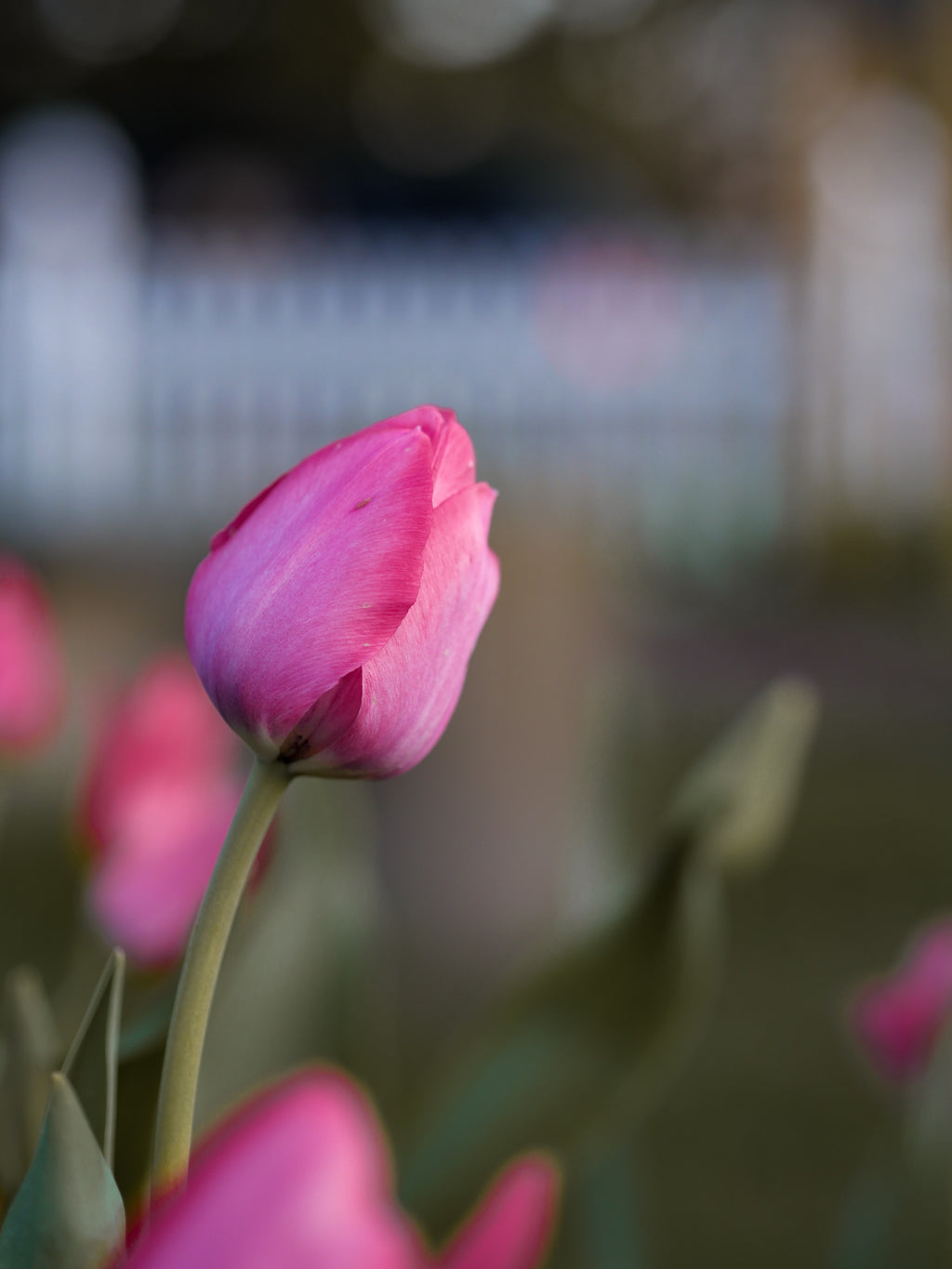The photograph is a high-resolution, vertically oriented rectangle featuring a photorealistic and beautifully detailed image of fuchsia or pink tulips in the foreground. These tulips, which haven't fully bloomed yet, are supported by vibrant green stems. There are six tulips arranged prominently and sharply focused in the center of the image. The background showcases a blurred, bokeh effect consisting of a white fence, green foliage, and other flowers, enhancing the depth of field. The lighting is subtly darker in the background, which accentuates the brightly lit tulips, creating a striking focal point in what appears to be a serene garden setting.